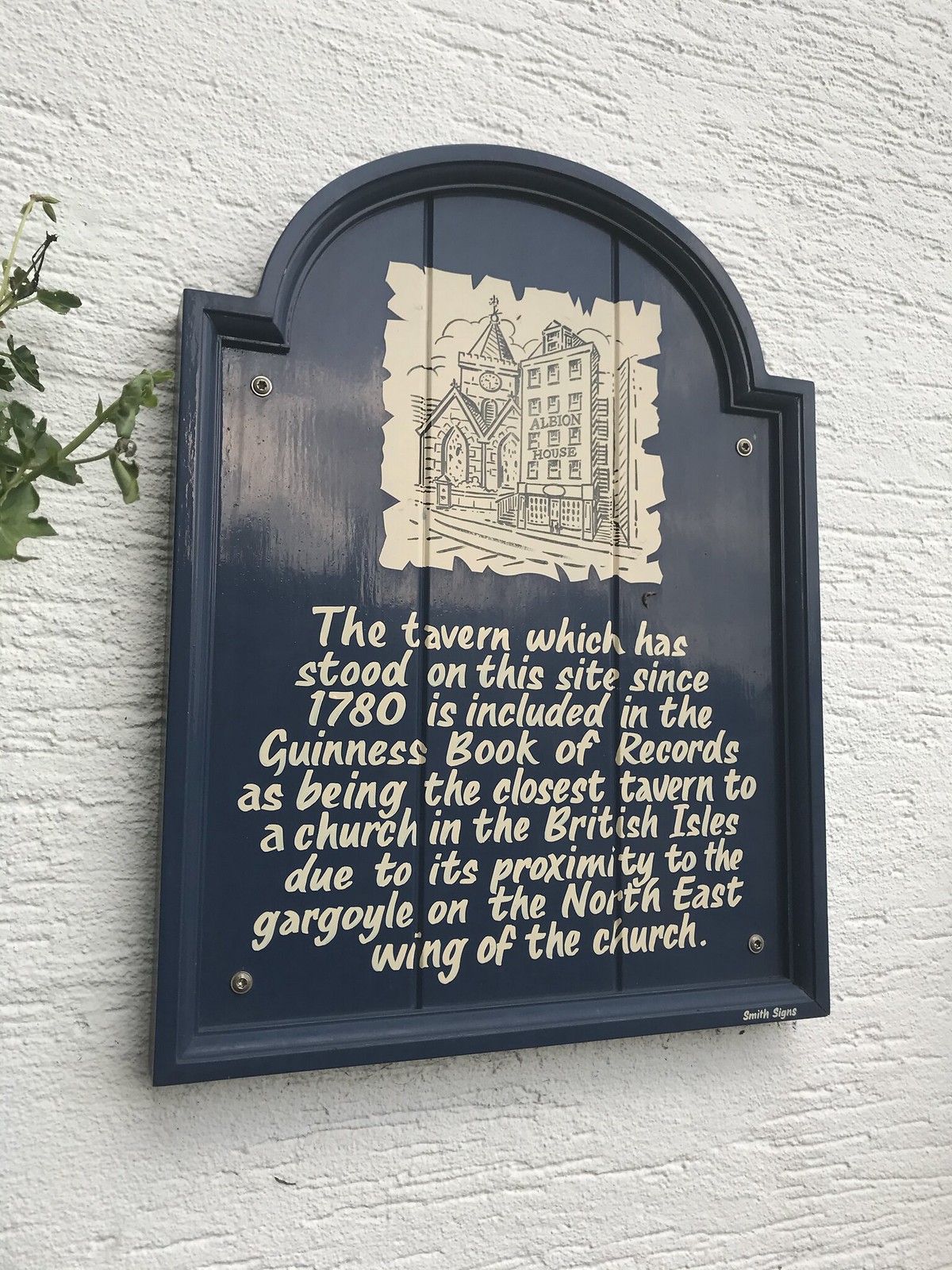The historical plaque featured in the color outdoor daylight photograph is mounted on a whitewashed, rough stone wall. There is green foliage protruding from the left side of the image. The plaque itself, painted blue and constructed from three pieces of wood with a curved top, is affixed to the wall via silver bolts at each of its four corners. At the top of the plaque, an artistic drawing depicts a medieval scene, prominently featuring the Albion House tavern and a nearby church, both labeled accordingly. Below the illustration, written in a gold, handwritten font against a beige background designed to resemble torn paper, the plaque details: "The tavern which has stood on this site since 1780 is included in the Guinness Book of Records as being the closest tavern to a church in the British Isles due to its proximity to the gargoyle on the northeast wing of the church." At the very bottom right corner of the plaque, there is small text identifying the maker, "Smith Signs."